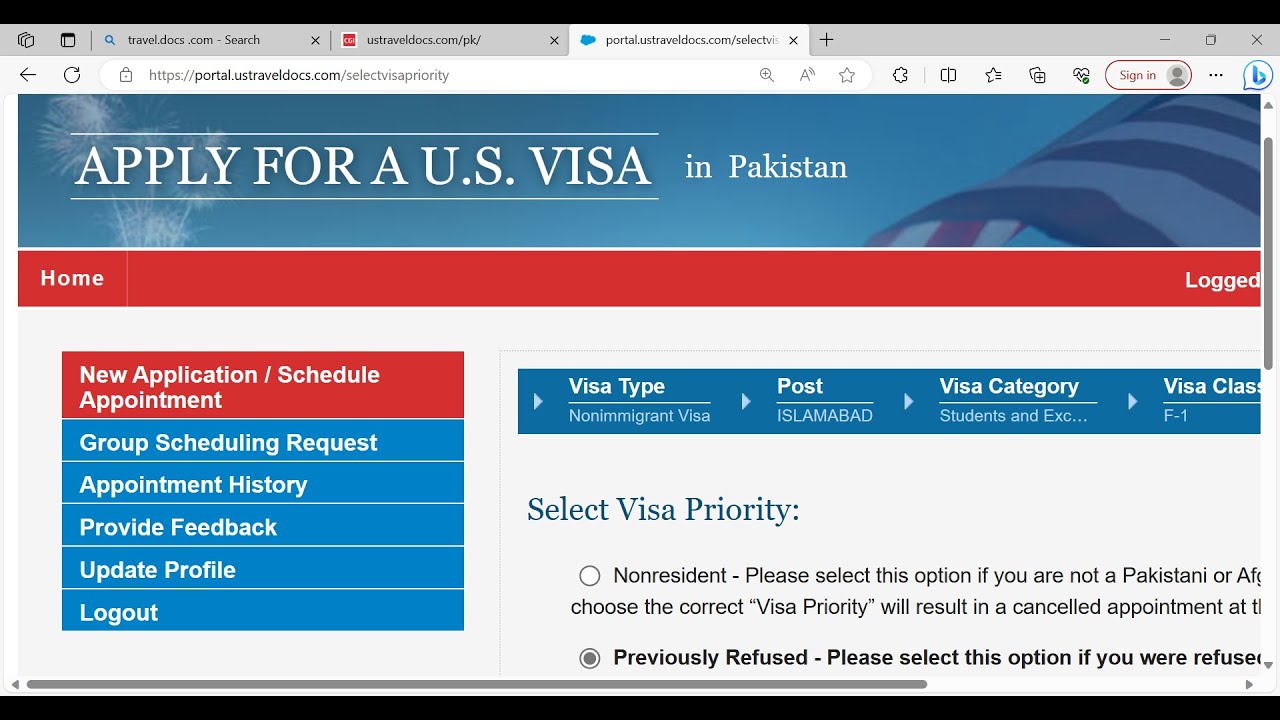This rectangular image, oriented with its longer sides extending from left to right, is framed by a thin black border at the top and bottom. The image appears to be a screenshot captured within a web browser window, showcasing three open tabs. The first tab reads "traveldocs.com," the second "traveldocs.com/pk," and the third "portal US travel docs."

In the active tab, a prominent blue-bordered section prominently displays the text "Apply for a US Visa in Pakistan" in white. Beneath this is a red-bordered header bar with the word "Home" in white at the far left and "Logged" at the far right.

As we move further down the image, we encounter a vertical menu on the left-hand side, featuring a variety of options in colored boxes. The top option, "New Application/Schedule Appointment," is presented in a red box with white text, while the remaining options—"Group Scheduling Request," "Appointment History," "Provide Feedback," "Update Profile," and "Log Out"—are in blue boxes with white text.

To the right of this menu, there is a blue box displaying visa application progress details. It indicates the "Visa Type" as "Non-immigrant Visa" with a directional arrow pointing to the right towards "Post: Islamabad."